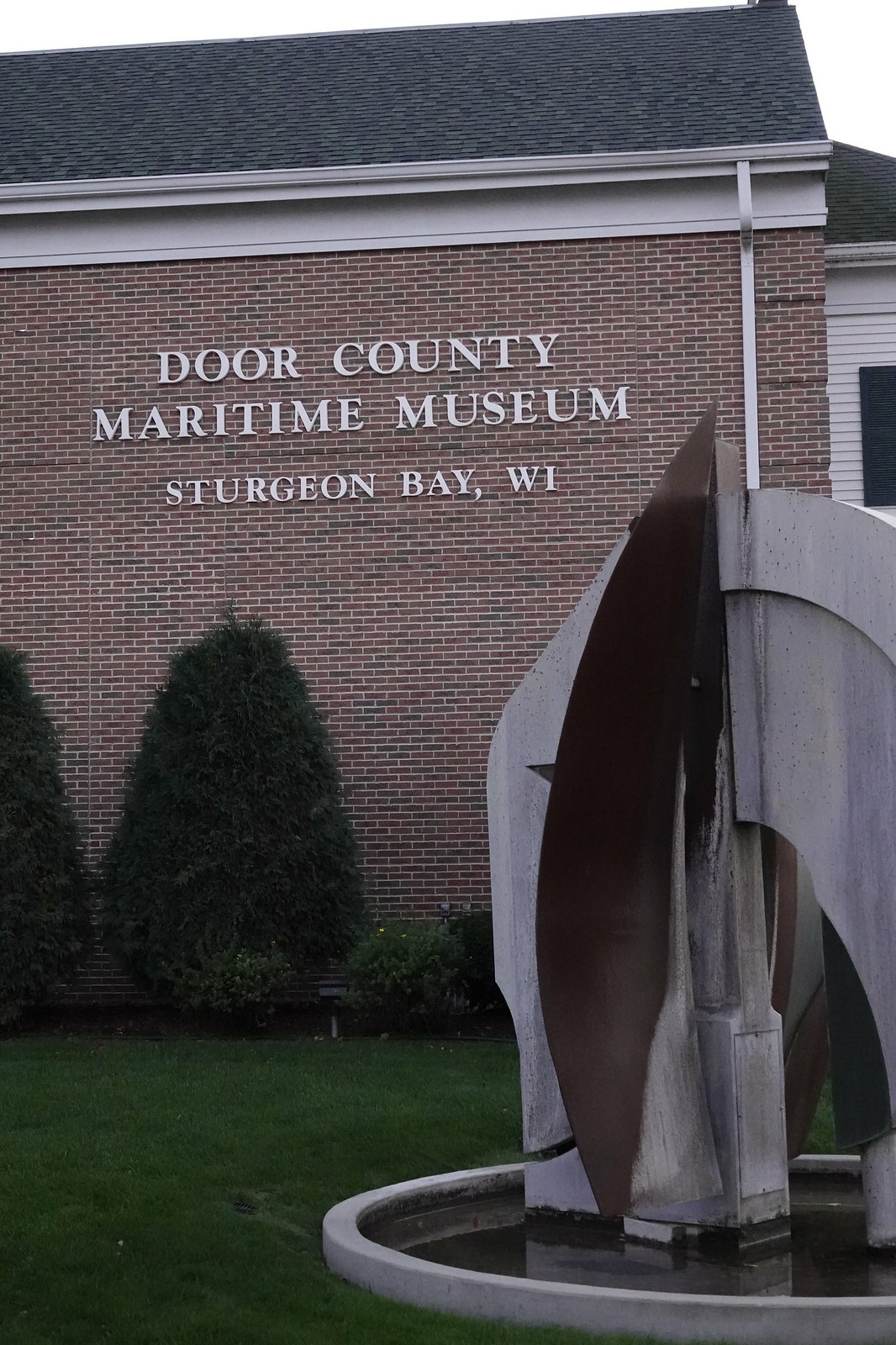The photograph captures the exterior of the Door County Maritime Museum in Sturgeon Bay, Wisconsin. The museum is housed in a tall, red brick building with a dark gray shingled, angled roof. Prominently displayed on the side of the building are white letters that read: "Door County Maritime Museum, Sturgeon Bay, Wisconsin". 

In front of the brick wall, there is an array of green bushes, including oval-shaped and coniferous types, contributing to the well-manicured setting. The foreground features a lush green grass field, and to the right of the image, there is an intriguing stone sculpture. This art piece is set in a circular stone base that contains a shallow amount of water, giving it the appearance of a small pond. The sculpture itself is composed of geometric shapes, with a combination of white and dark brown colors resembling a knife blade on the left and a half-circle on the right.

The photo was taken during the day under an overcast, white sky, adding a soft light to the scene. The overall composition highlights both the architectural and artistic aspects of this notable museum.